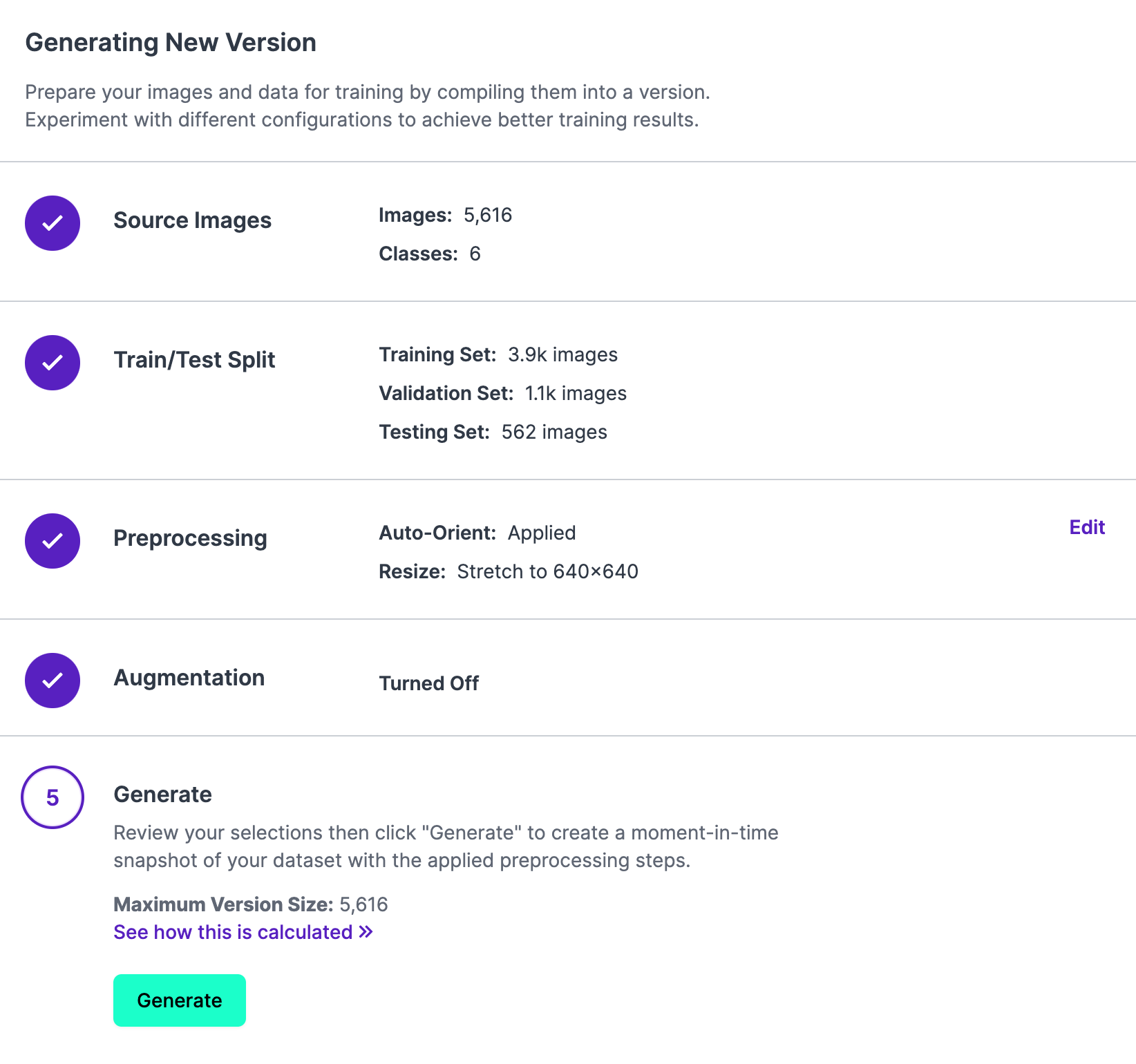The image displays a screen with the heading "Generating New Version." Below this, instructional text reads: "Prepare your images and data for training by compiling them into a version. Experiment with different configurations to achieve better training results." 

On the left side, there are five sections listed in sequence, each preceded by a purple circle. The first four sections – Source Images, Train-Test Split, Preprocessing, and Augmentation – have already been checked off. The current step, Generate, is highlighted. 

Additional guidance instructs users to review their selections and then click "Generate" to create a snapshot of their dataset with the applied preprocessing steps. It notes that the maximum version size is 5,616, with a clickable purple link offering an explanation of how this size is calculated.

At the bottom of the screen, there is an aqua-colored button labeled "Generate" for users to click and proceed.